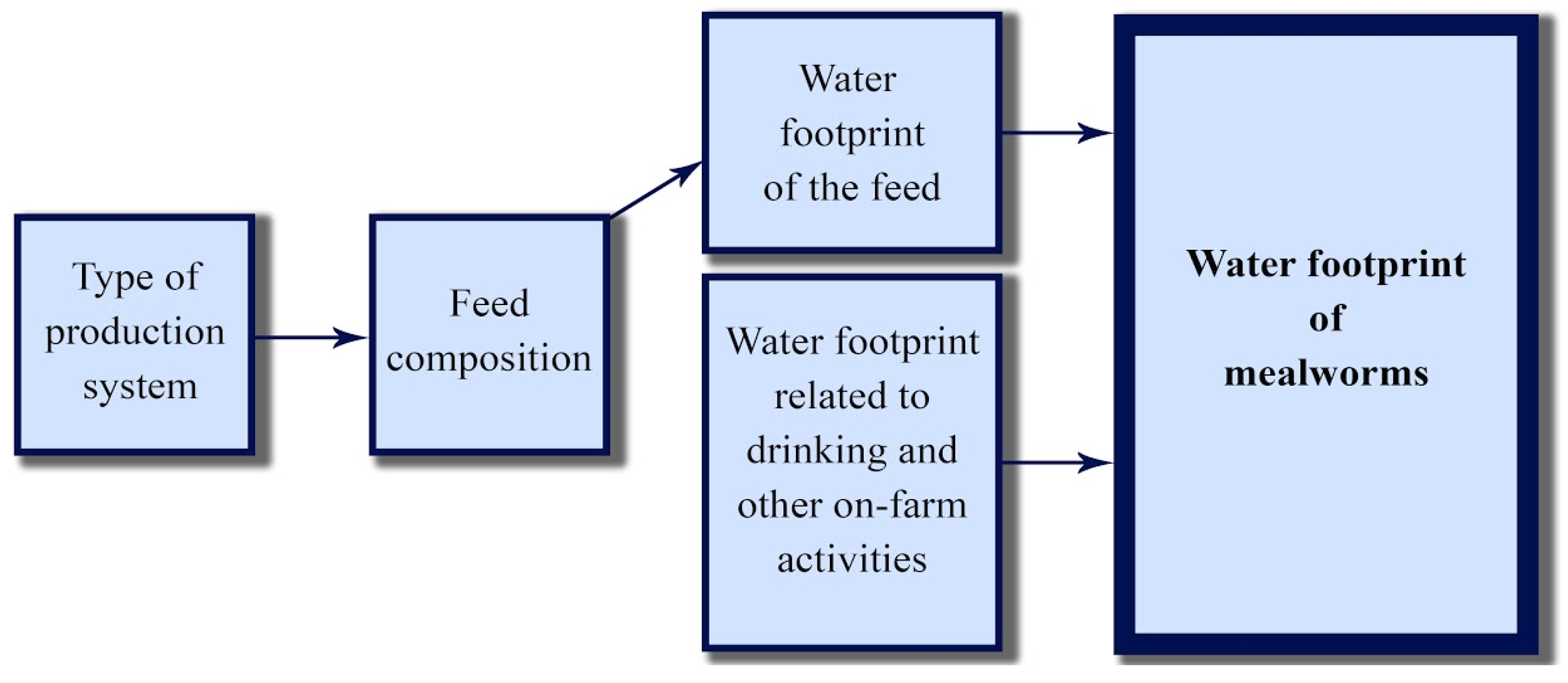The image depicts a detailed landscape-oriented flowchart focused on mealworm production and its associated water footprint. The chart is composed of several light blue boxes with dark blue borders and black text. Starting from the left, the first box is labeled "Type of Production System," which is connected via an arrow to a box labeled "Feed Composition." An arrow extends from the top-right corner of this box diagonally upwards to a box labeled "Water Footprint of the Feed." Below this, horizontally aligned, is another box labeled "Water Footprint Related to Drinking and Other On-Farm Activities." Both of these boxes point to a larger, bolded rectangle on the right side labeled "Water Footprint of Mealworms." The flowchart illustrates the different components contributing to the overall water footprint in the production system of mealworms.